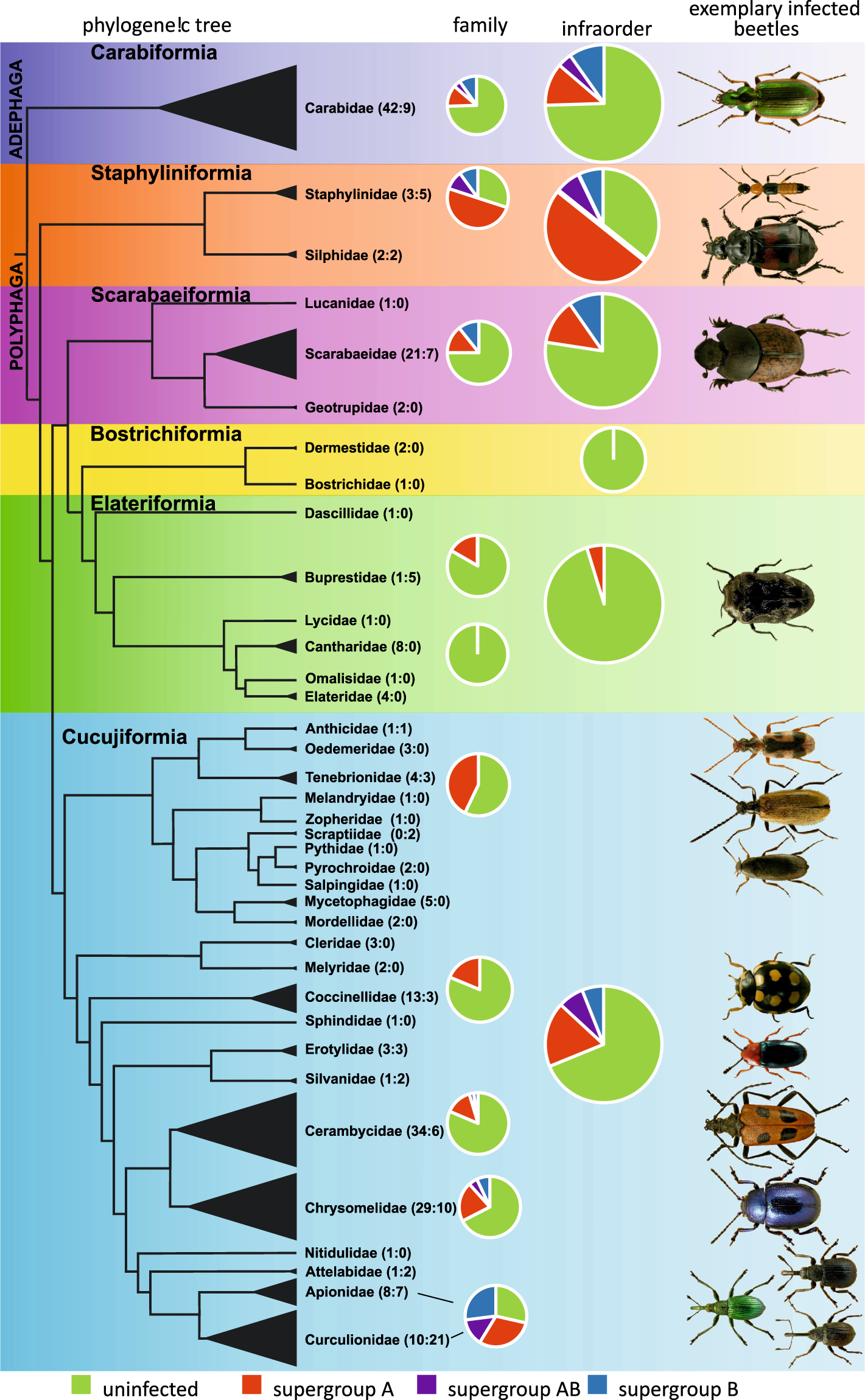The diagram illustrates various groups of beetles, segmented into a phylogenetic tree organized into four columns. Starting from the left, the columns are labeled as "Phylogenetic Tree," "Family," "Infra Order," and "Exemplary Infected Beetles." The "Phylogenetic Tree" column details the evolutionary lineage of numerous beetles, listing their scientific names comprehensively. Directly to the right, the "Family" column displays small pie charts colored in shades like blue, purple, red, and green, representing different beetle families. The "Infra Order" column also presents pie charts but on a larger scale, utilizing similar color schemes.

The rightmost column, "Exemplary Infected Beetles," showcases images of distinct beetle species exemplifying various infections. Each section of the phylogenetic tree is color-coded: the largest section at the bottom is light blue, followed by a light green section, a smaller yellow section, then purple, orange, and dark blue sections ascending upwards.

At the top, the classifications in each column assist in understanding the relational structure of beetle families, infra orders, and infections highlighted with specific visual aids. The key at the bottom explains the color codes: green indicates uninfected beetles, red represents Super Group A, purple signifies either Super Group B or AB, and blue denotes Super Group B.